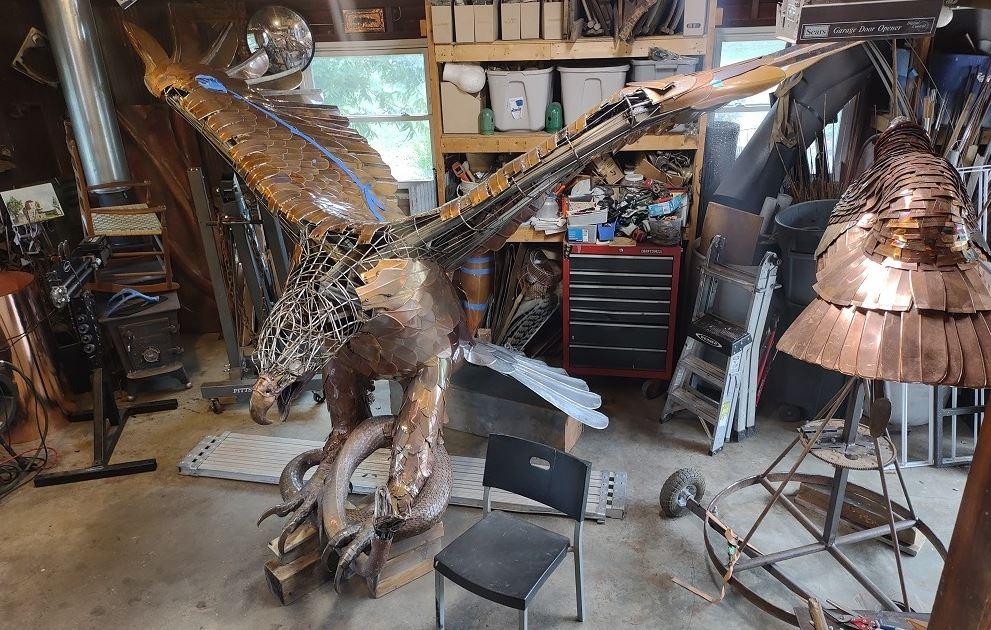In a bustling metalworking garage filled with various tools, supplies, and a background of miscellaneous objects including ladders, bins, and shelving units, two intricate bronze sculptures dominate the scene. The centerpiece is a partially completed, chrome-plated statue of a majestic eagle with its wings majestically spread and its powerful talons coiled around a snake, seemingly in battle. The eagle's body and wings are meticulously crafted, though the head and neck areas are yet to be covered with metal, revealing the wire frame beneath. Adjacent to it stands another sculpture, possibly depicting a tail or a different creature, partially obscured and turned away from the viewer. The concrete floor, scattered with materials and a chair likely used by the artist, emphasizes the ongoing creation process in this workshop adorned with windows and full of creative energy.